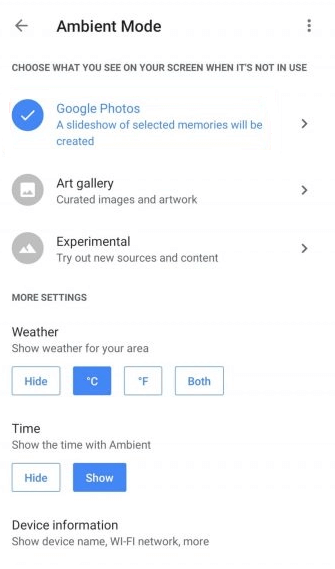This screenshot captures the Ambient Mode settings menu on a mobile device. At the top, the heading reads "Ambient Mode," followed by the instruction: "Choose what you see on your screen when it's not in use." Beneath this, three options are presented: "Google Photos," "Art Gallery," and "Experimental," with "Google Photos" currently selected. Further down, there is an option for additional settings, such as toggling the display of weather or time. At the bottom of the screenshot, a section titled "Device Information" appears, likely offering details about the device and its ambient mode functionality.